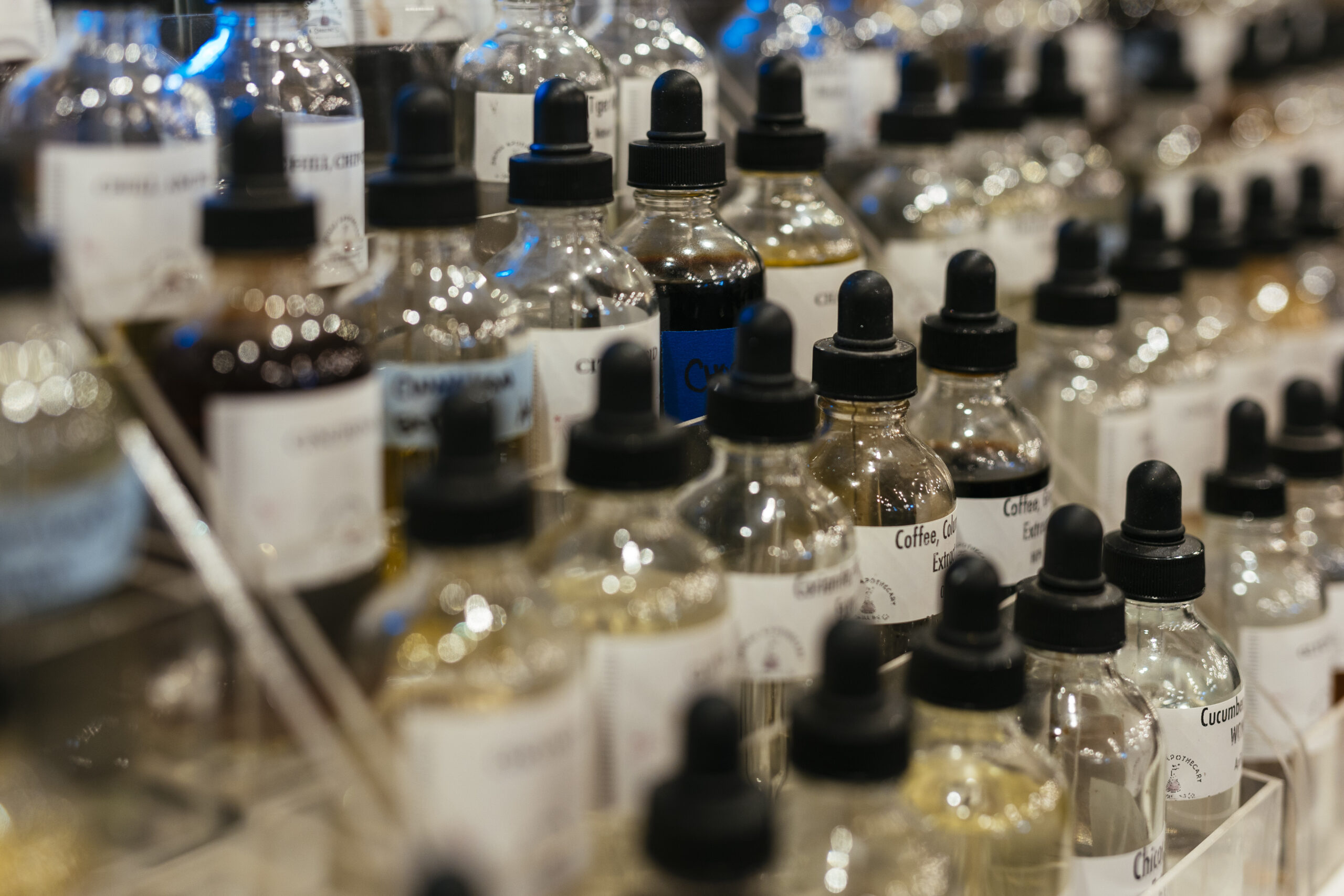This color photograph features multiple rows of clear glass dropper bottles, each topped with black plastic droppers. The bottles are arranged closely together, creating an impression of being in a container or on a display platform, with some rows positioned on a higher level in the background. The bottles' reflective surfaces capture light, adding a shimmering effect to the image.

Most of the bottles are adorned with white labels, although a few distinct labels can be noted: one in the center that prominently displays "coffee" and another that might indicate "cucumber." Additionally, there is one bottle with a striking blue label.

The background rows appear blurry and out of focus, making the text on those labels difficult to read. The overall arrangement and varying label details suggest that these bottles could be used for holding coffee flavors or other liquid extracts.